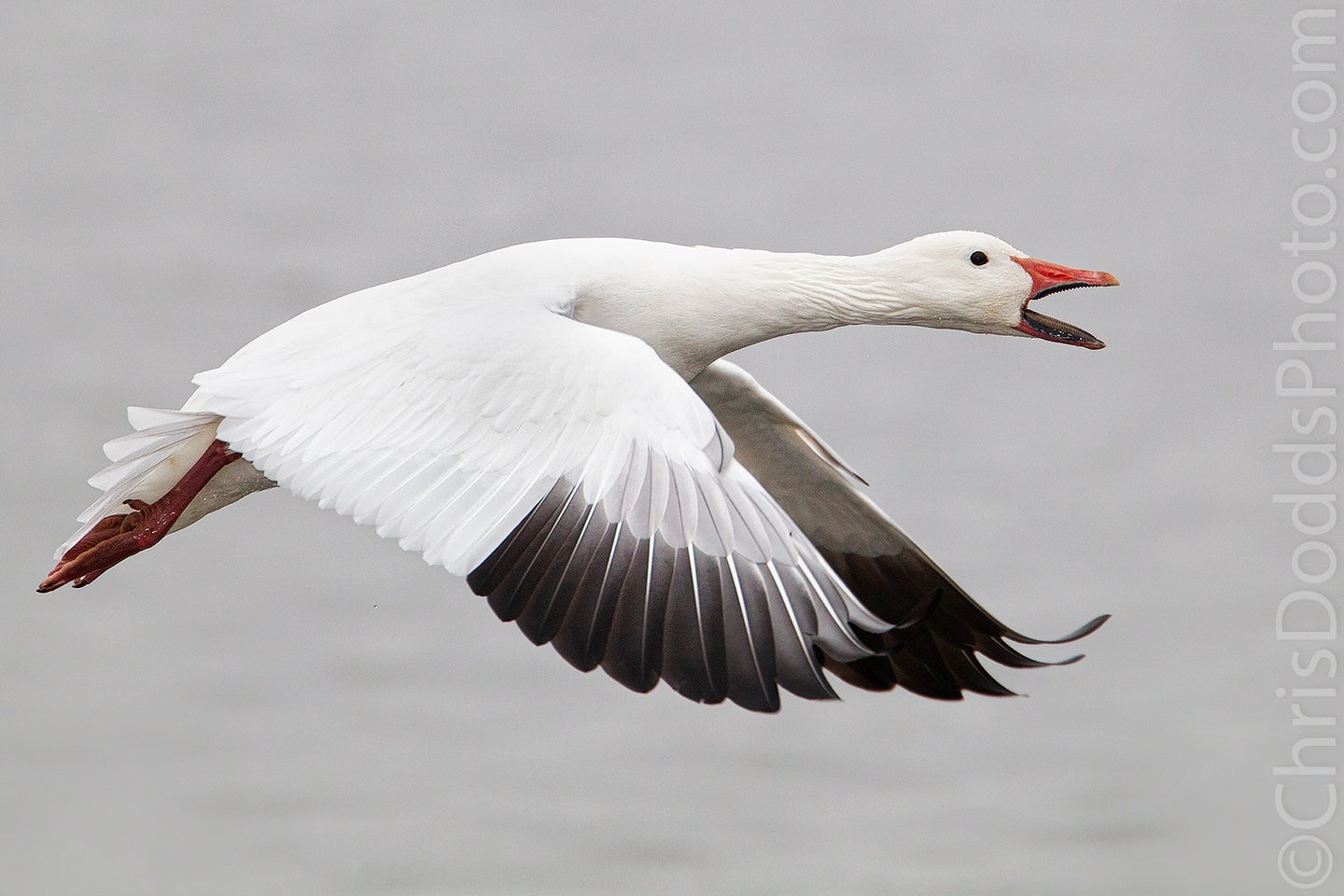This detailed photograph captures a stunning close-up of a white geese bird in mid-flight, prominently displaying its black-tipped wings, vivid red beak, and small black eye. The bird, shown with its wings down and mouth open, adds a dynamic sense of motion. Its red legs are visible under the wings, trailing behind as it soars. The backdrop features a calm, gray expanse of water, possibly an ocean or lake, slightly out of focus to emphasize the bird's clarity. The image is a fine example of nature photography, credited with the watermark "chrisdoddsphoto.com" appearing on the right side of the frame.